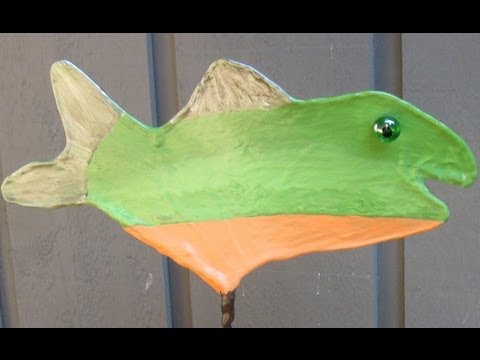The image captures a handmade fish sculpture mounted on a metal rod against a gray paneled wall. The fish, which appears to be crafted by a child, is oriented with its head pointing to the right. It has a vibrant green body with an open mouth, and a glass eyeball that is green with a black pupil. The fish's top and bottom fins are white, while the bottom part of the fish is a striking yellow-orange, and the tail is also white. The background reveals three vertical slats on the gray wall, suggesting an indoor setting possibly made from plaster. The fish exudes a childlike charm and creativity, showcasing a whimsical piece of tangible artwork.